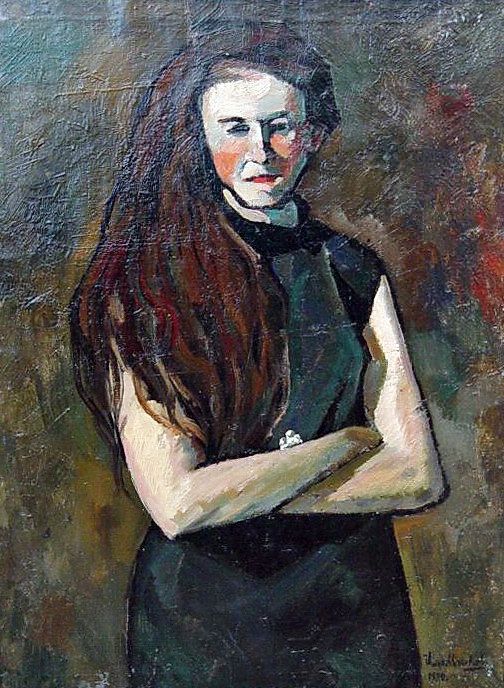The image is an oil painting that seems to be of a modern, albeit slightly abstract, depiction of a woman. The central figure is a pale female, with long hair that varies in description from brown to red, cascading down past her shoulders. She stands upright, her arms crossed beneath her breasts, and is dressed in a dark, short-sleeved gown that appears either dark blue, dark purple, or black. Her expression is somewhat ambiguous, possibly conveying anger, focus, disapproval, or foreboding, with slightly squinting eyes. Her cheeks are distinctly orange, contrasting with her very white, pale skin. The background is a dull array of rusty reds, browns, and other muted colors, blending flatly with the figure, giving a unified, plane-like appearance. There's an illegible signature in the bottom right corner of the vertical rectangular painting.